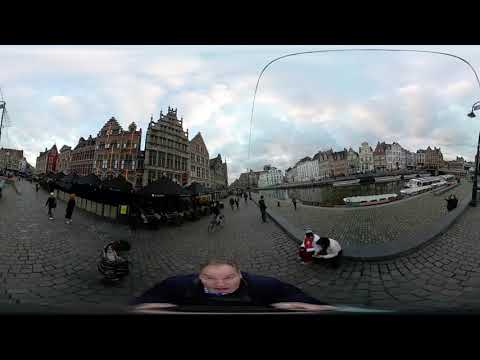In the image, a fisheye distortion creates an intriguing visual effect, most notably on a gentleman positioned prominently in the front. This man, wearing a black or blue shirt, appears significantly widened due to the camera's effect, and his hands are visible but heavily distorted. He has thin brown hair and is balding. The street he's standing on is paved with dark, possibly reddish to deep gray bricks, indicative of a historic or European cityscape, reminiscent of the Netherlands with its old, stone-front buildings painted in white, light gray, and lighter red. These buildings are adorned with triangular, pointed roofs.

The background is bustling with activity. There is a brick walkway or street where several people are seen from behind: two individuals to the left are walking, and another person is riding a bike. To the right and slightly behind the main figure, two people, dressed in white but heavily distorted, are sitting on a curb or low stone wall. In the upper right-hand side of the photo, a body of water is visible with some white boats resting on the dark, almost black-looking water. The surrounding scene is captured under a cloudy sky, adding to the historical ambiance of the setting.